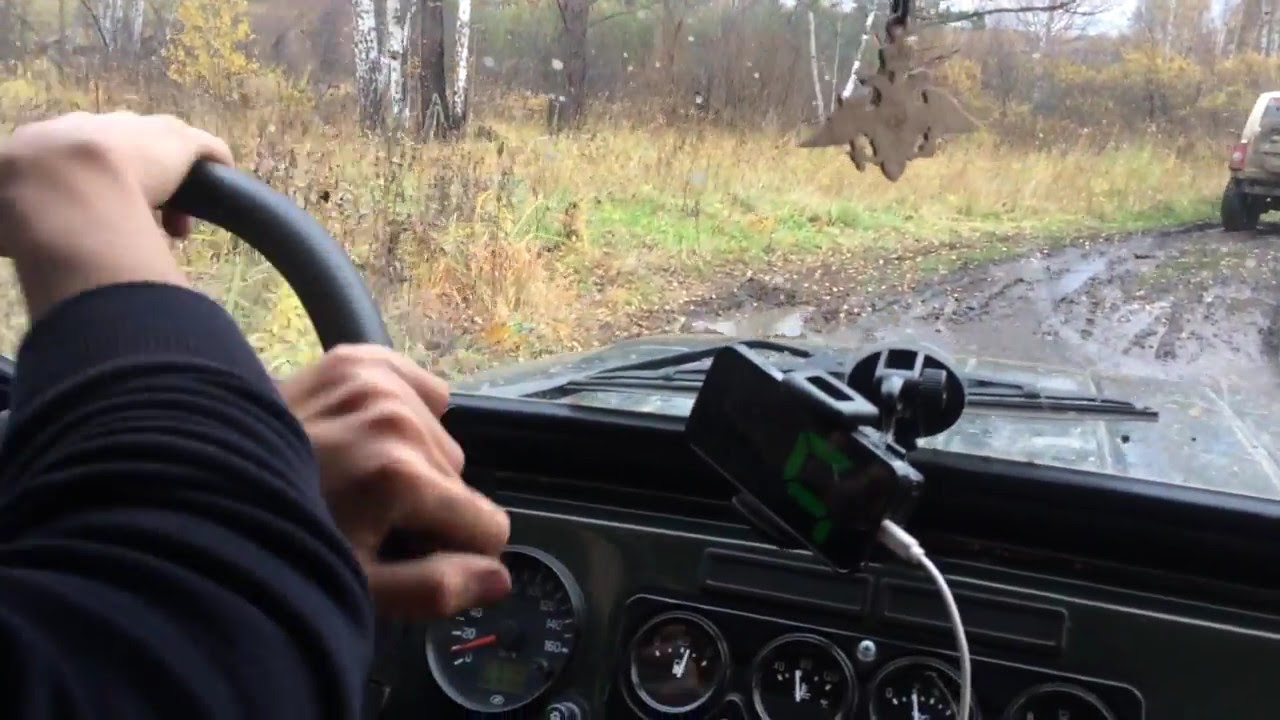This photograph captures the perspective from inside a car, focusing on a person driving down a muddy, wet road. The driver’s hands, with a medium skin tone, grip the black steering wheel, and they are wearing a long-sleeved black shirt. The dashboard is visible, showing the speedometer and other gauges. An object resembling wings or possibly an eagle hangs down, likely from the rearview mirror. Through the car's windshield, the muddy, unpaved road takes a right turn, and a partially visible Jeep can be seen exiting the frame on the top right, revealing only its back left wheel. The road appears wet and muddy, indicating rainy conditions. On the left side outside the car, there's a mix of green and brown grass and scattered trees, adding to the scene’s rugged, natural environment.